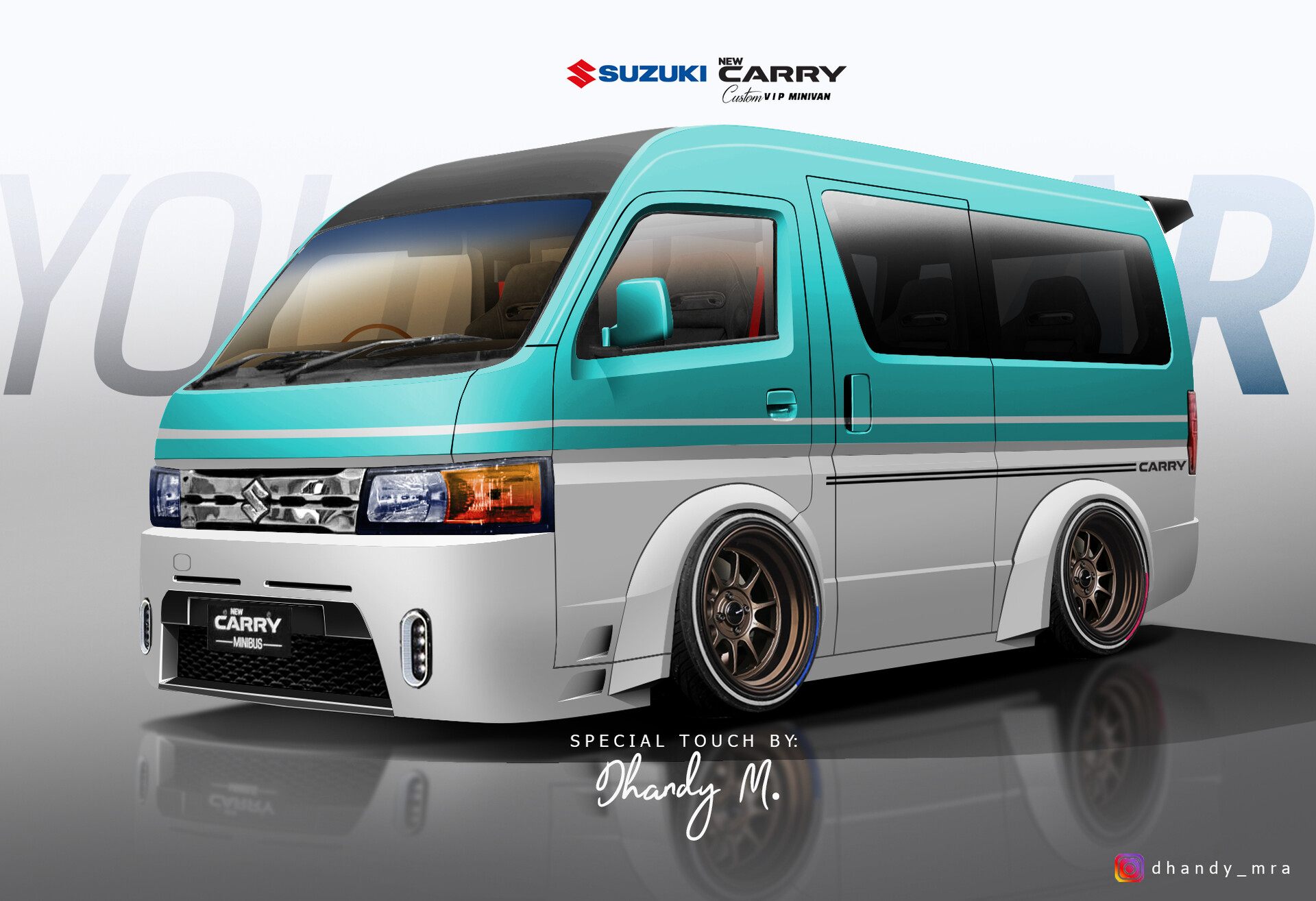This Instagram image from user @dandy_MRA showcases a digital rendering of the futuristic Suzuki New Carry VIP minivan. The stylish vehicle boasts a sleek two-tone color scheme with a white lower half and a turquoise blue upper section, accentuated by black pinstriping. It sits low to the ground, sporting eye-catching copper-colored rims and low-profile tires. The design includes a flat front and a highly sloped, almost futuristic-looking windshield. The minivan's windows, possibly tenon, suggest it has two to three rows of seats behind the driver. The floor beneath the vehicle is a reflective gray, enhancing the high-tech vibe. Text in the background, though partly obscured by the van, includes letters like Y, O, and R, and the words "Special Touch by Dandy M." are noted at the bottom of the image. The entire image is digitally created, emphasizing the modern design concepts rather than a real-world photograph.